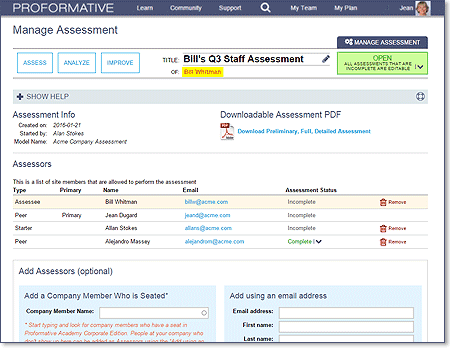**Caption:** 

The screen displays an internal company management or assessment interface. At the top, there's a dark purplish-blue toolbar that reads "PRO-FORMATIVE" in all caps white lettering. Adjacent to this are options: "Learn," "Community," "Support," a magnifying glass icon for search, "My Team," and "My Plan." On the far right, there's a profile picture of a Caucasian woman with bob-cut blondish hair, labeled "Jean."

The main background of the screen is white with the heading "Manage Assessment" in black text. A black line stretches almost the entire width of the screen, ending with the blue tab reading "Manage Assessment" again. Below this, there are three options in light blue text boxes labeled "Assess," "Analyze," and "Improve."

The title "Bulls Q3 Staff Assessment" and the name "Bull Whitman" are prominently displayed. A "Show Help" option is available, though small, as well as assessment details dated January 21, 2016. Users can download the assessment as a PDF.

Below this, a section lists the assessors with their email addresses in light blue text. The names listed include Bull Whitman, Jean Ugard, Alan Stokes, and Alejandro Messi. Only Alejandro has completed his assessment, indicated by an apparent status next to his name; the others have incomplete assessments. There's also an option to remove assessments.